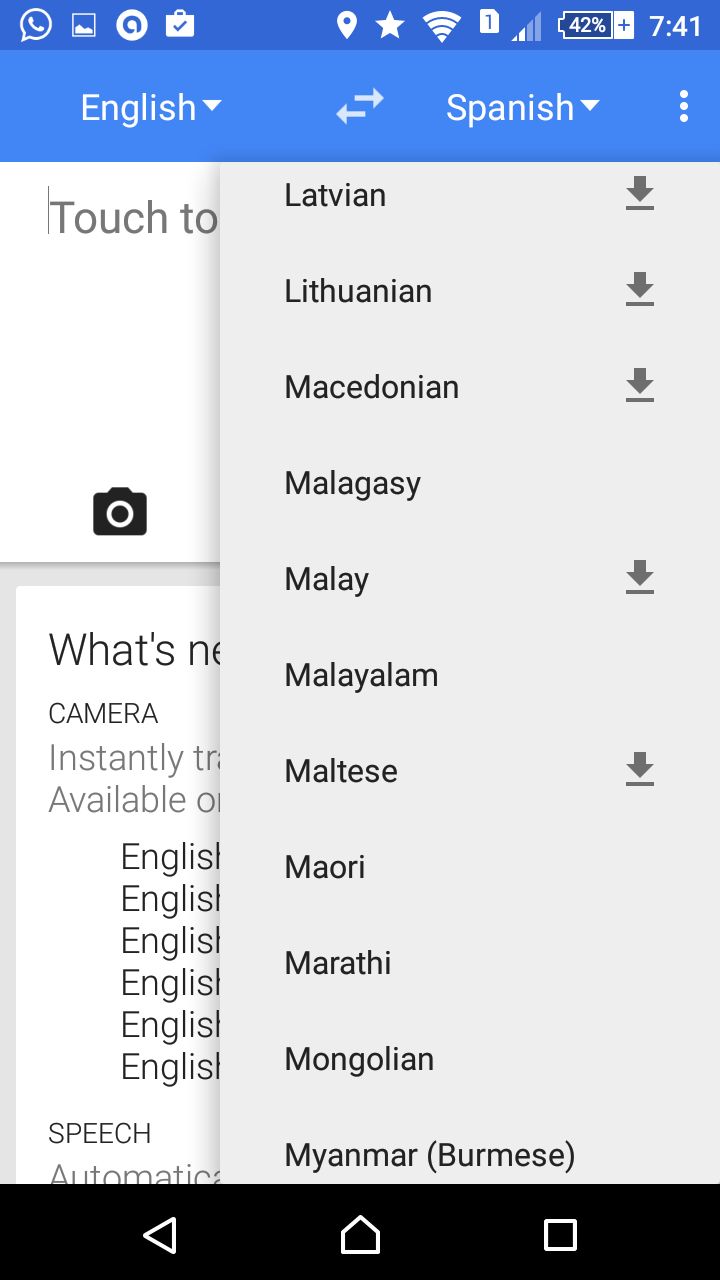This is a screenshot from a mobile phone. At the top of the screen, there is a blue status bar displaying various icons. The battery level is at 42%, there are two bars of network coverage out of four, and the Wi-Fi signal is at full strength with four bars. Below the status bar, an app is visible that translates English to other languages. English is set as the source language, and Spanish is chosen as the target language. There is an expanded menu showing other languages that English can be translated into, such as Latvian, Lithuanian, Macedonian, Malagasy, Malay, Malayalam, Maltese, Maori, Marathi, Mongolian, and Myanmar (Burmese). However, only five of these languages display a download symbol, indicating that translations to some of the languages are unavailable for offline use. In the background, partially obscured by the language menu, is an icon of a camera.